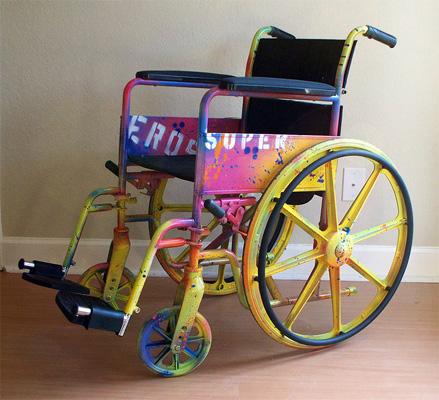This is an indoor photograph, taken in a square format of approximately three inches by three inches. The background of the image features a light tannish white wall with a white baseboard occupying the top two-thirds, while the lower third consists of light brown wood flooring. At the center of the scene is an unoccupied wheelchair facing to the left. The wheelchair is a vivid kaleidoscope of colors, primarily adorned with shades of pink, yellow, bluish-purple speckles, and hints of green, creating an interactive and graffiti-like appearance. The backrest, seat, footrests, armrests, and handle grips of the wheelchair are black, providing a stark contrast to the colorful frame. The wheel rims remain black, while the wheels themselves display yellow paint with splashes of graffiti-like purples and blues. Notably, the word "Super" is spray-painted on the outer side of the wheelchair, and "E-R-O-S" appears in white on the inside, although the latter is somewhat obscured. The setting includes details like an outlet on the wall, helping to emphasize the indoor environment.